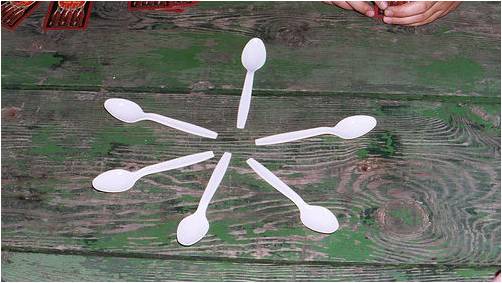The photograph captures a daytime scene of a worn, natural wood picnic table, with remnants of faded green paint. Viewers have an overhead perspective, revealing clear wood grain textures and slight green patches, suggesting previous paint or moss. A striking arrangement of six clean, white plastic spoons forms a flower-like starburst pattern at the center, with spoon heads facing outward and handles inward, creating an empty circle in the middle. The spoons are evenly spaced and aligned symmetrically. In the upper right corner, partial hands are visible, fingers lightly touching the table, hinting at a casual, outdoor setting. The upper left corner inadvertently includes some indistinguishable objects, possibly playing cards. The image is in clear focus, emphasizing the details of both the spoons and the aged picnic table.